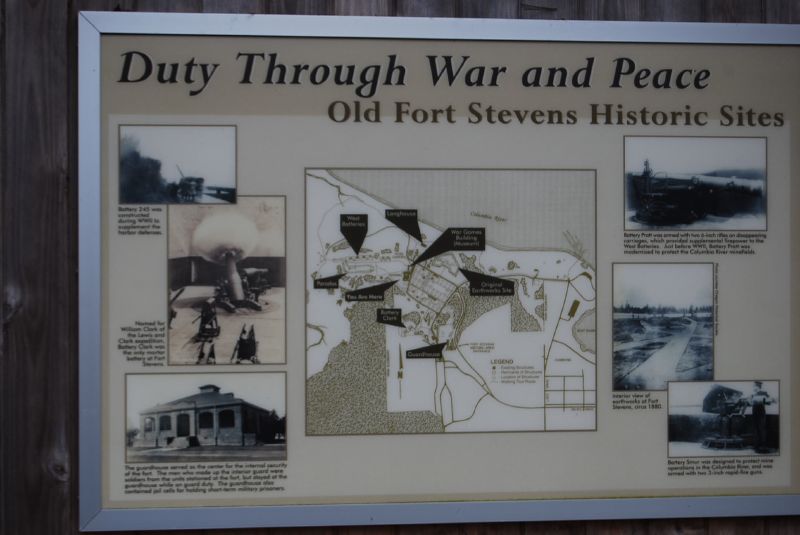This image depicts a framed sign mounted on a wooden paneled wall, likely at a museum or historic site. The centerpiece of the image is a sign with a metal border that reads "Duty Through War and Peace, Old Fort Stevens Historic Sites." The sign includes a central map showing various historic sites, marked by arrows. Surrounding the map, on both the left and right sides, are black and white photographs. On the left, the pictures include a fort, a steam engine, and a cannon with a cannonball. On the right, the images include a road, an unidentified object, and a piece of historical machinery. Despite small and hard-to-read text scattered across the sign, the primary focus is on visual portrayals of historical elements and sites related to Old Fort Stevens. The colors in the image are mostly natural tones, including gray, brown, tan, white, black, and yellow, complementing the wooden and metallic textures. The overall setting suggests this sign provides an informative glimpse into the historical landscape and activities associated with Fort Stevens.